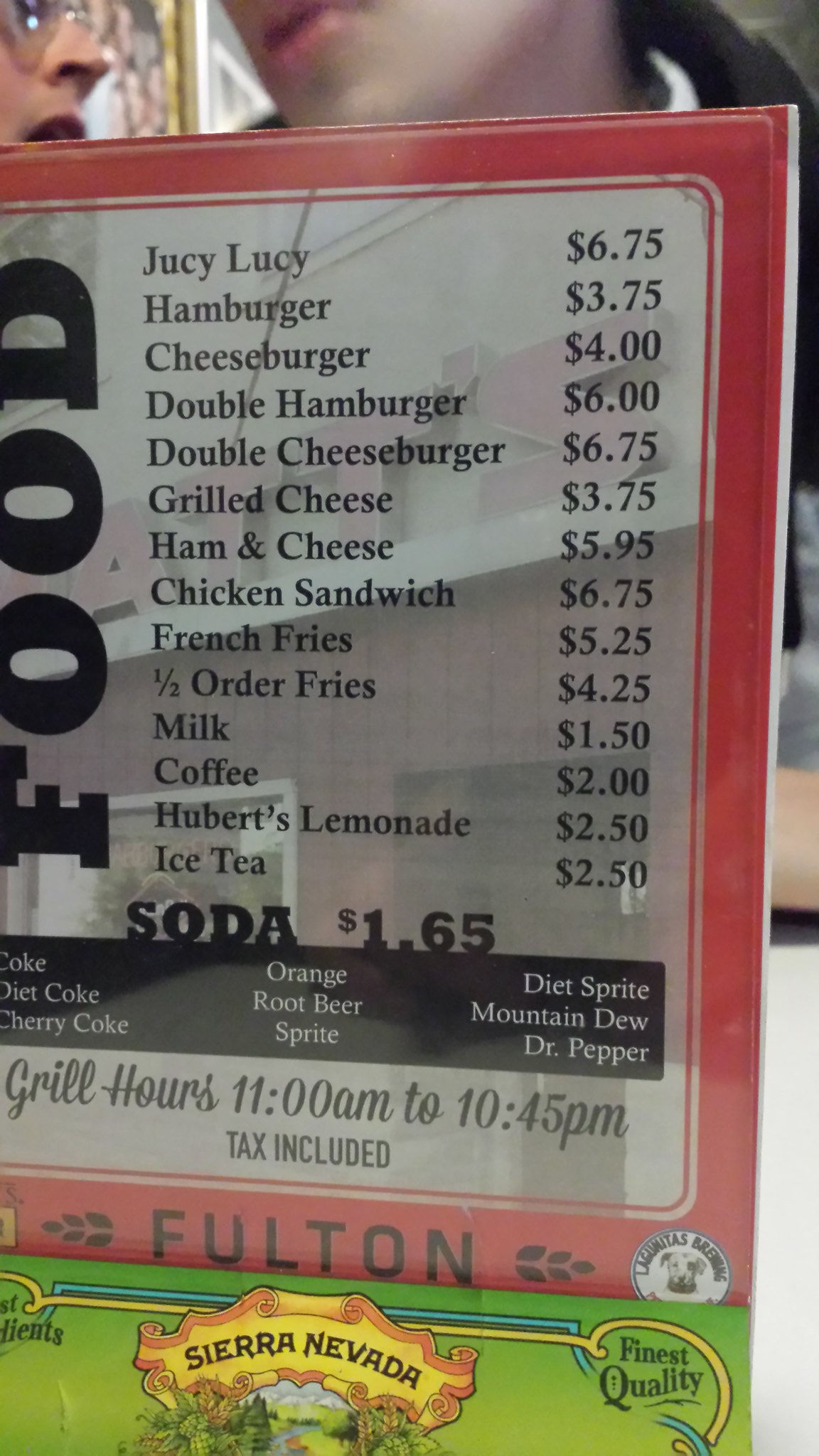In this photograph, a paper menu is prominently displayed standing upright inside a clear plastic frame attached to a stand. Behind the menu, there is a man visible from the nose down, dressed in a white shirt and a black jacket, engaged in conversation with another individual whose eyes, nose, and mouth are partially visible.

The menu itself is white with a distinct red border, and the establishment's name, "Fulton," is printed at the bottom. Running along the side in bold black letters is the word "FOOD." The menu features a vertical list of various food items including:

- Juicy Lucy
- Hamburger
- Cheeseburger
- Double Hamburger
- Double Cheeseburger
- Grilled Cheese
- Ham and Cheese
- Chicken Sandwich
- French Fries
- Half Order Fries
- Milk
- Coffee
- Hubert's Lemonade
- Iced Tea
- Soda

Beneath this list, a black banner provides details about the available soft drink options. Below the banner, on the white portion of the menu, "Grill Hours" are specified as 11 a.m. to 10:45 p.m., along with a note indicating that tax is included in the prices. At the very bottom, there is a lime green section displaying the Sierra Nevada logo and a small inscription that reads "Finest Quality" in the corner.